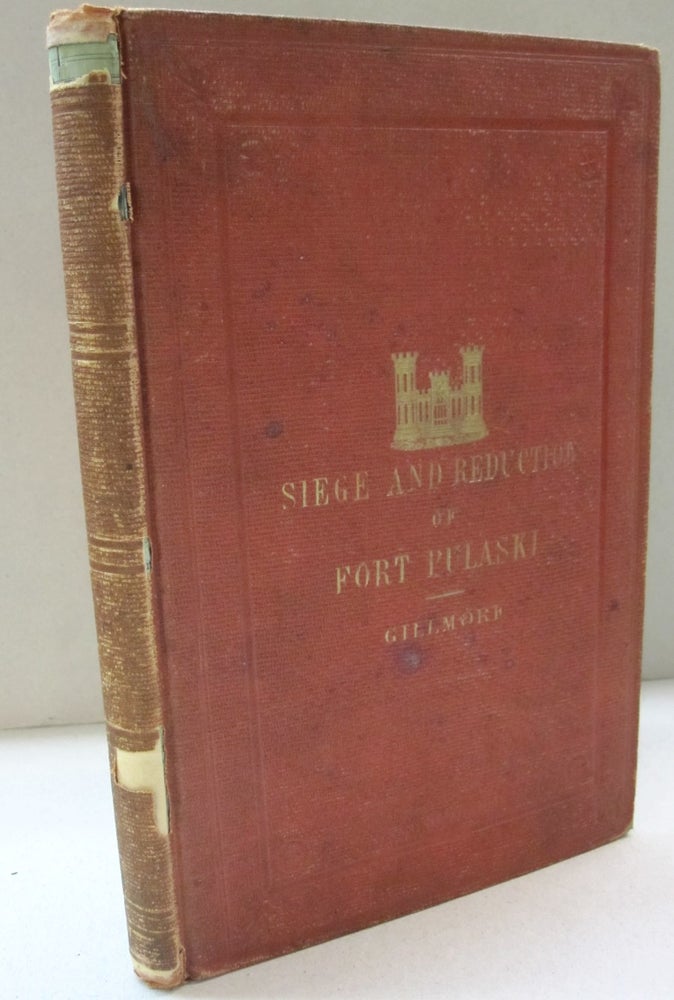This photograph features a worn, fabric-bound hardcover book with a predominantly faded red cover and a brown, tattered spine. The book stands upright on a white surface against a white wall, casting a slight shadow that lends the wall a grayish hue. The cover of the book is adorned with a faded gold-embossed image of a castle with two towers, likely representing the contents of the book. Below this image, in gold lettering, is the title "Siege and Reduction of Fort Pulaski," and beneath that, the author's name "Gilmore." The condition of the book is quite poor; parts of the fabric on the spine have stripped away, especially near the top, revealing the white and light green binding material underneath. Stains mar the front cover, emphasizing the book's age and wear. The perspective of the photo shows the spine along the left side, and the book itself appears slightly slanted.